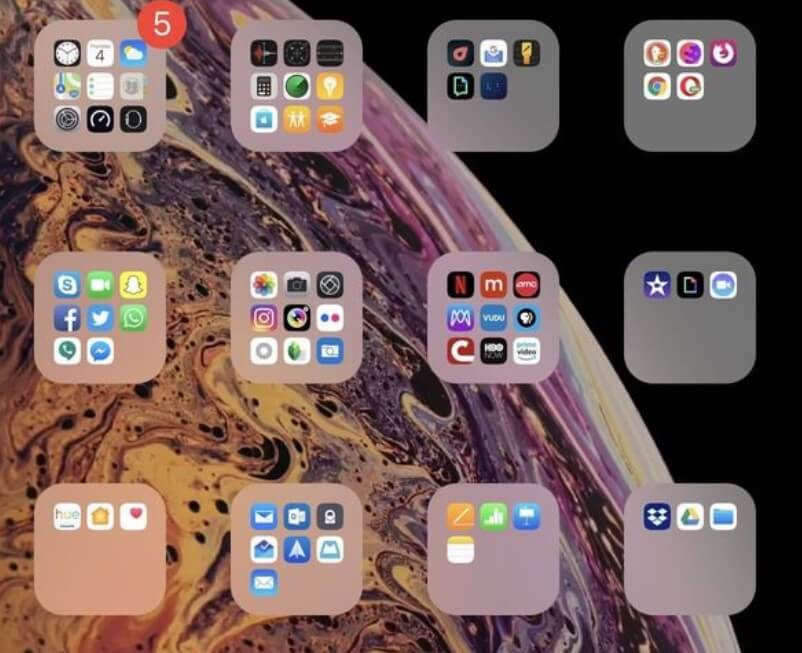The image features a striking composition with a black background on the right side, and a vivid, swirling depiction of a planet on the left side. The planet is adorned with a dynamic mix of purple, yellow, black, and gray swirls, resembling a marbled painting. To the right of the planet are 12 evenly arranged squares, each containing various phone app icons.

Among the squares, a red circle with a white number "5" is positioned slightly to the right. Each square contains a distinct app icon, beginning with a clock in the top left, which has a white face, black hands, and a black border. Next to it, there's a space displaying the date "4" in white on a blue background, accompanied by a sun partially obscured by a white cloud. 

The subsequent row includes a map, a notes app icon, and a gray placeholder. Below these, the settings icon is showcased, featuring a white gear with black accents. Adjacent to this is a timer icon with a white center and black outline, and an app icon that is likely for the Apple Fit Watch. Other icons within the grid include those for Netflix, a camera, Microsoft apps, and several nondescript placeholders, all set against the consistent gray backgrounds of the squares.

The overall image blends vibrant planetary artistry with a structured, orderly arrangement of everyday digital icons, merging the cosmic and the mundane.